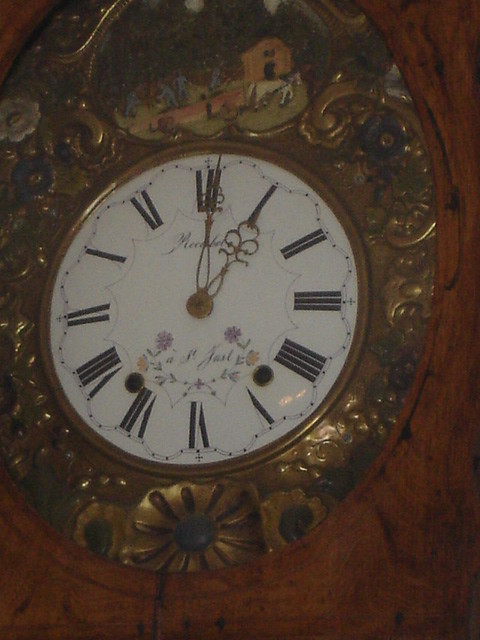The image showcases an antique, analog clock set into a dark, wooden wall. The clock features a white face adorned with black Roman numerals, with intricately designed gold hands shaped like delicate floral patterns. Surrounding the clock face is a lush border of wreaths and crosses, meticulously crafted from brass and featuring detailed floral engravings. The base of the clock extends into the wood, culminating in a gold flower design at the bottom. At the top of the clock, a charming painting depicts a pastoral farm scene with a horse pulling a plow, a farmer working beside it, and a barn in the distance. This timeless piece, with its blend of utility and refined artistry, captures the essence of early 20th-century craftsmanship.